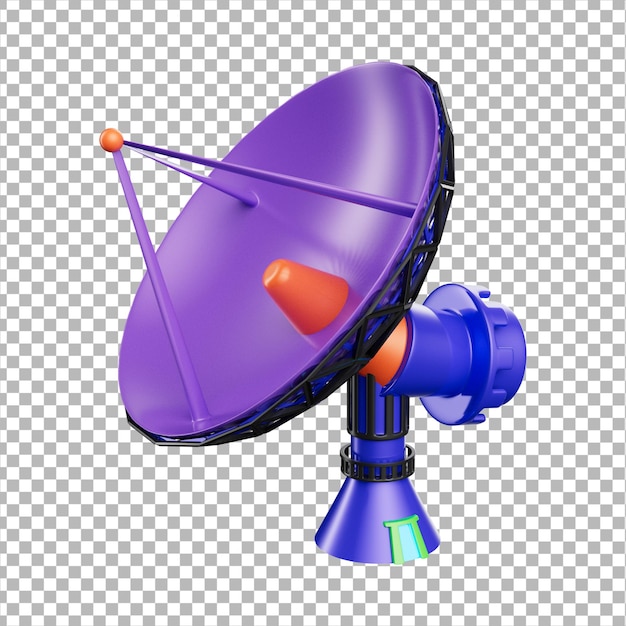The image features a toy satellite dish set against a checkered, white and gray background designed to ensure transparency. The dish part of the satellite is a lighter shade of purple, while the base connector is a darker purple. The dish is intricately fashioned with triangular, pipe-like structures that converge at a small orange ball at the top. An orange cone sits at the center of the dish, appearing to wedge it in place. The base, which is designed to hold the satellite up, is blue with a turning mechanism to simulate old-fashioned satellite dishes that could rotate to receive TV channels. Additional details include black crisscrossed bars around the perimeter of the dish, a green button or connector at the bottom, some black structural framework, and hints of light blue at the base.